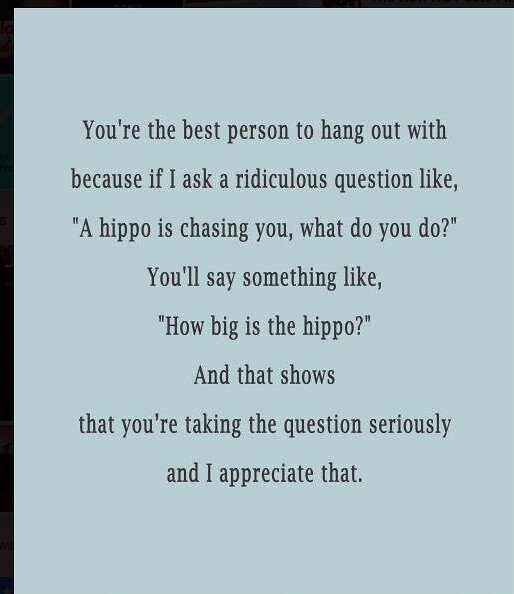The image features an inspirational quote set against a light blue-gray background with a black border running along the top and left side, the left border being thicker than the top. The only colors visible in the image are the light blue-gray background, the black borders, and the black text. The quote is centered both horizontally and vertically and reads: "You're the best person to hang out with. Because if I ask a ridiculous question like, 'A hippo is chasing you, what do you do?' you'll say something like, 'How big is the hippo?' and that shows you're taking the question seriously. I appreciate that." The font is typical and plain, with the text spanning from about 15% to 85% of the vertical length of the image. There are no other elements, people, or colors in the image, making the focus solely on the message conveyed by the quote.